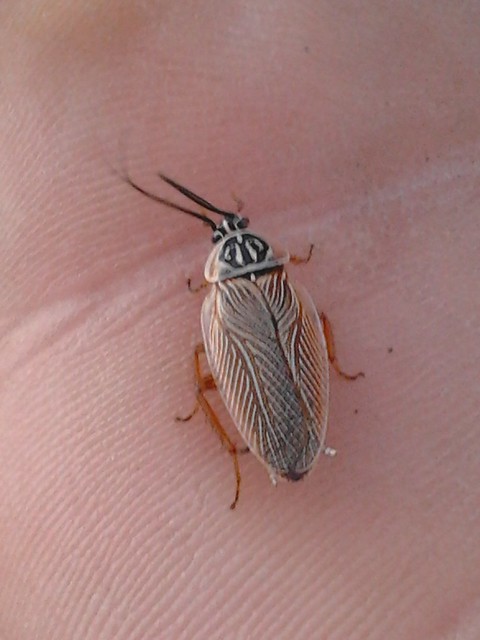The image is a close-up of a vibrant, multicolored beetle resting on the slightly dried skin of a person's hand. The beetle features a striking combination of brown, black, and white hues, with elegant black antennae protruding from its head. Its body displays brown, black, and white stripes on its wings, while the head showcases a white base adorned with a black design, and black eyes. The beetle is positioned on a light brown area of the hand, providing a stark contrast against the light pink background observed in other parts of the image. The fine ridges and a line running through the center of the hand are visible, emphasizing the detailed texture of the skin. The beetle stands out prominently, particularly its intricately patterned head, making the image a fascinating display of natural detail. There is no text or writing present, allowing full focus on the beetle and the hand.